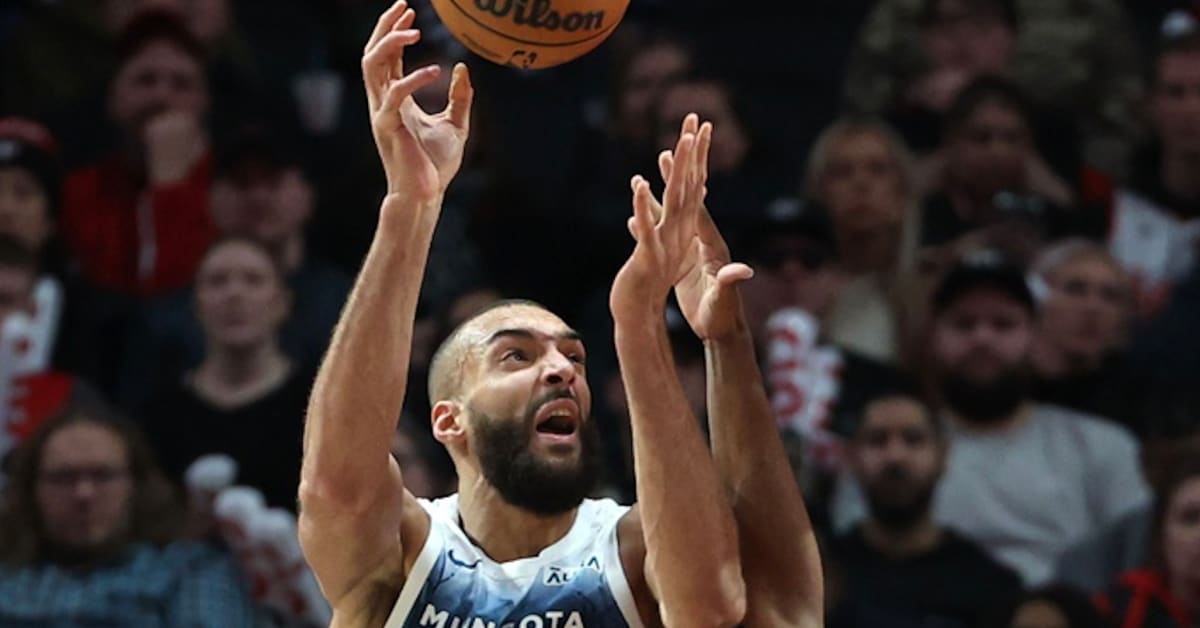In this dynamic and action-packed close-up photograph, we see a black basketball player, captured mid-game, from the armpits up. He has a light brown skin tone, a bald head, and a thick black beard and mustache. His mouth is open in anticipation as he looks up towards the top right corner of the frame. He is wearing a white jersey with blue trim, marked with an 'M' at the beginning of the team's name, and both of his arms are extended upwards. Just out of reach of his right hand is a brown basketball with the black logo "Wilson" prominently displayed, seemingly descending towards him. A third arm, protruding from the bottom of the frame, appears to be making an attempt to swat or block the basketball. The background reveals a blurred crowd of spectators seated in bleachers or a stadium, all intently focused on the action unfolding before them. Among the crowd, some members are holding white cups, and distinct figures include a man on the lower left wearing glasses and a blue shirt, and another man in the right corner with a beard and a black shirt.